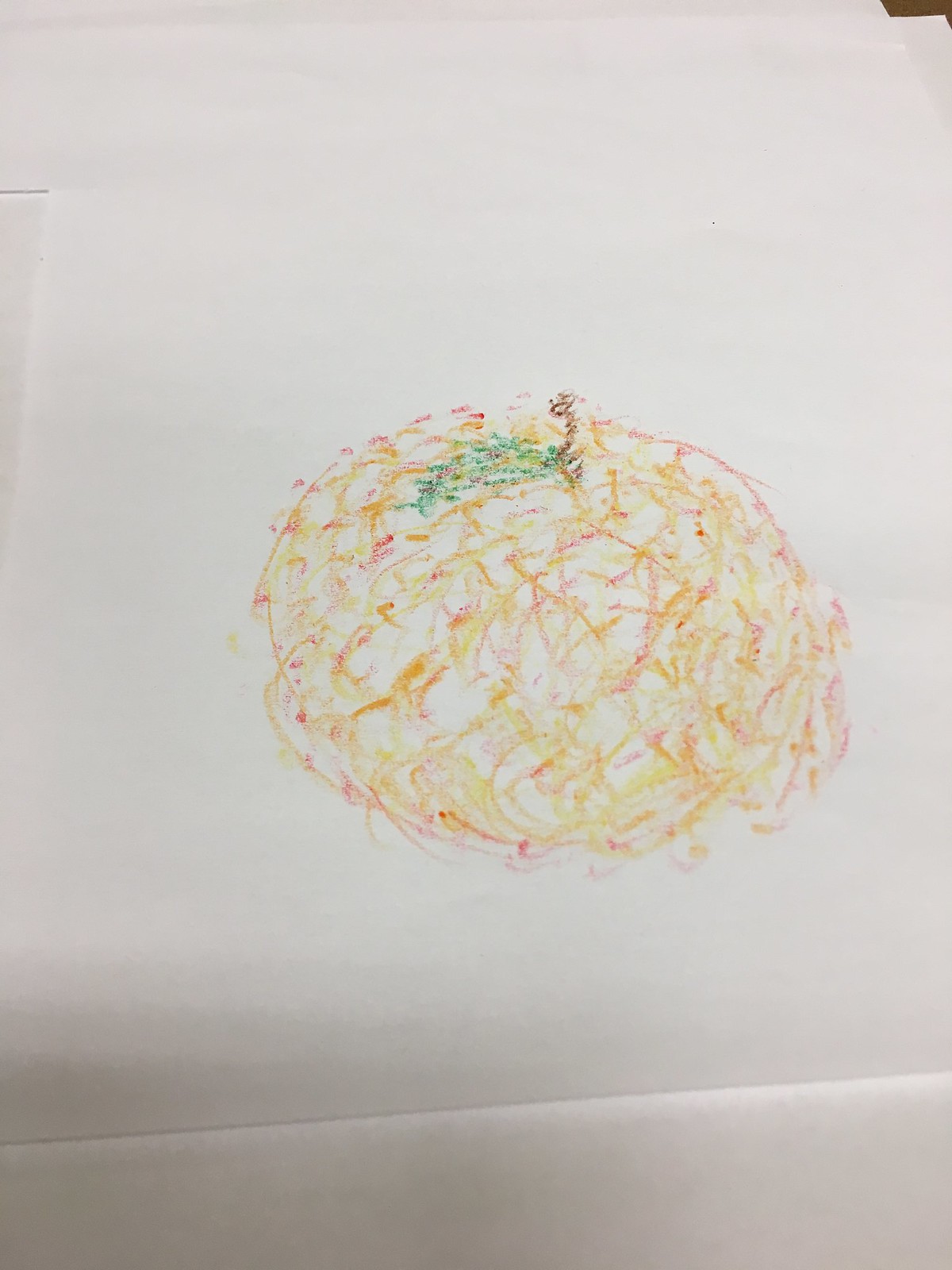This is a photograph capturing a hand-drawn image rendered in pencil on a white sheet of paper. Subtle creases are visible toward the bottom of the sheet, accompanied by some gray shadowing. A narrow sliver of a brown surface peeks from the top edge of the image. The drawing itself depicts a piece of fruit, combining hues of gold, yellow, and a faint red, with a brown stem and an abstract, scribbly green leaf. The image quality is crystal clear, showcasing no other illustrations on the paper. Additionally, some wrinkles are evident beneath the paper, suggesting multiple sheets are stacked together. The overall quality of the image is excellent.